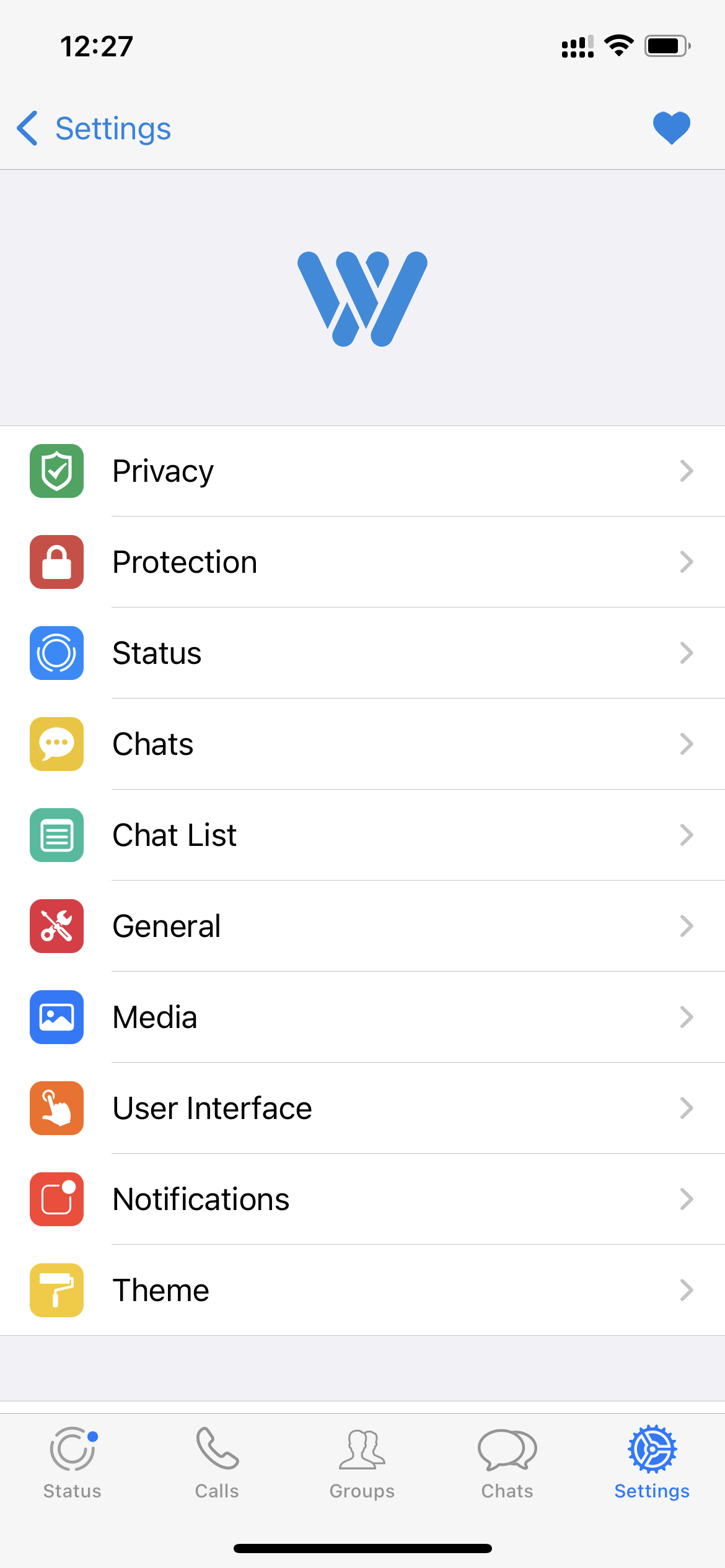A detailed screen capture of a smartphone showcasing the settings menu of an unidentified app. At the top of the screen, the time is displayed as 12:27, and the battery level is approximately 90-95% charged. The app's icon is prominently featured and consists of a blue "W" or "VV," designed with overlapping popsicle stick-like lines.

The settings menu is comprehensive, offering several options for customization and security. The listed categories are as follows: 
1. Privacy
2. Protection
3. Status
4. Chats
5. Chat list
6. General
7. Media
8. User Interface
9. Notifications
10. Theme

Additionally, at the bottom of the screen, navigation tabs are visible, which include: 
1. Status
2. Calls
3. Groups
4. Chats
5. Settings 

This capture provides a thorough glimpse into the app's extensive personalization and security features.